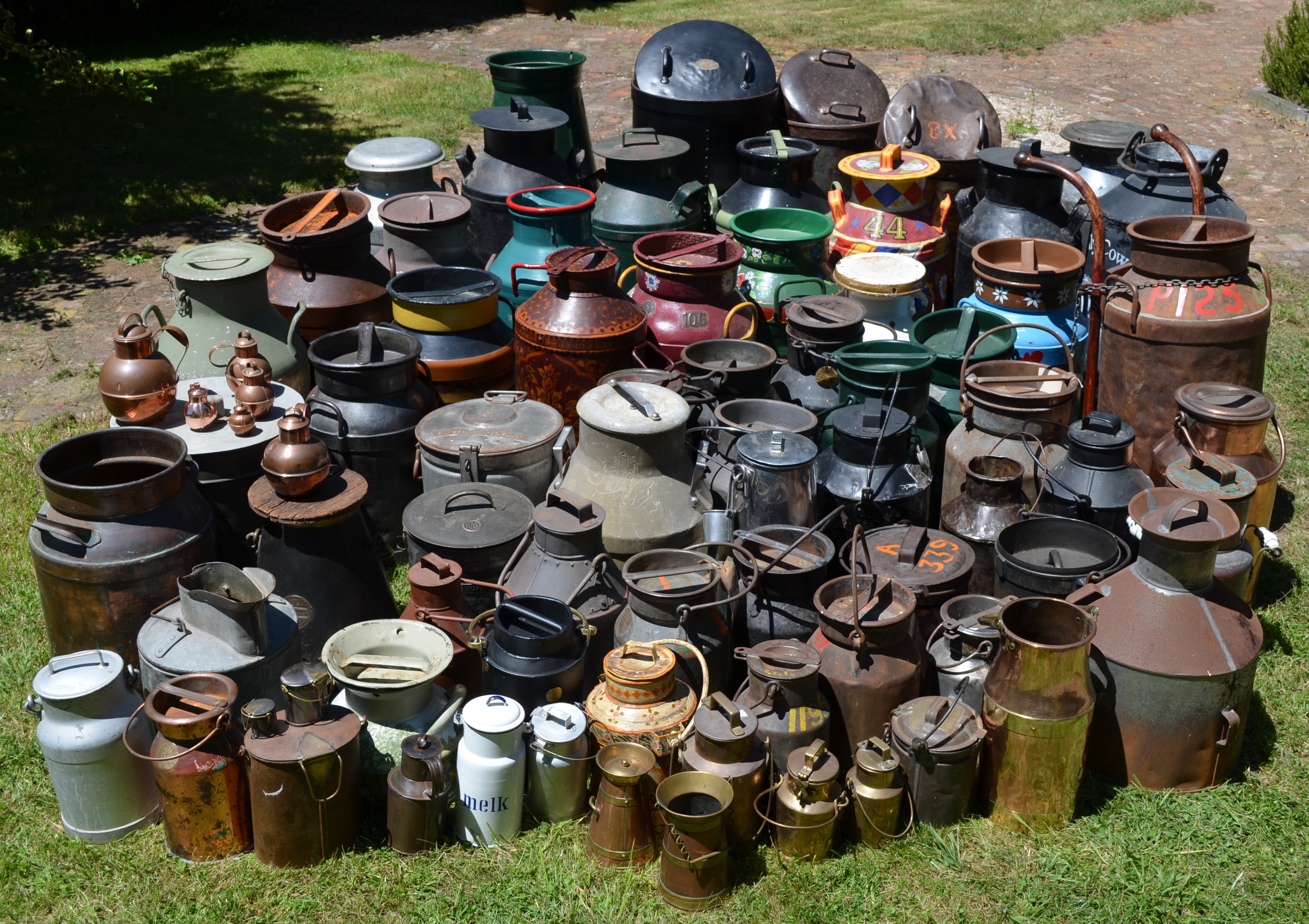This photograph captures an outdoor installation of approximately 100 to 150 vintage and antique milk jugs, containers, and spittoons, displayed in a circular arrangement on a grassy patch. The collection, meticulously ordered, features smaller containers in the front that gradually increase in size towards the back, some reaching the size of garbage cans or larger propane tanks. The containers, which vary in material from metal to possible bronze, boast a spectrum of colors including silver, gold, blue, green, and rust. While many have been painted, others remain plain or show heavy rust damage, giving them a weathered, antique appearance. The sunlit backdrop of grass and a brick stone walkway adds to the charm, suggesting this might be an artistic display or possibly items for sale. Among the assortment, there are standout details like a white jug with "m-e-l-k" painted on it, emphasizing the collection's vintage vibe.